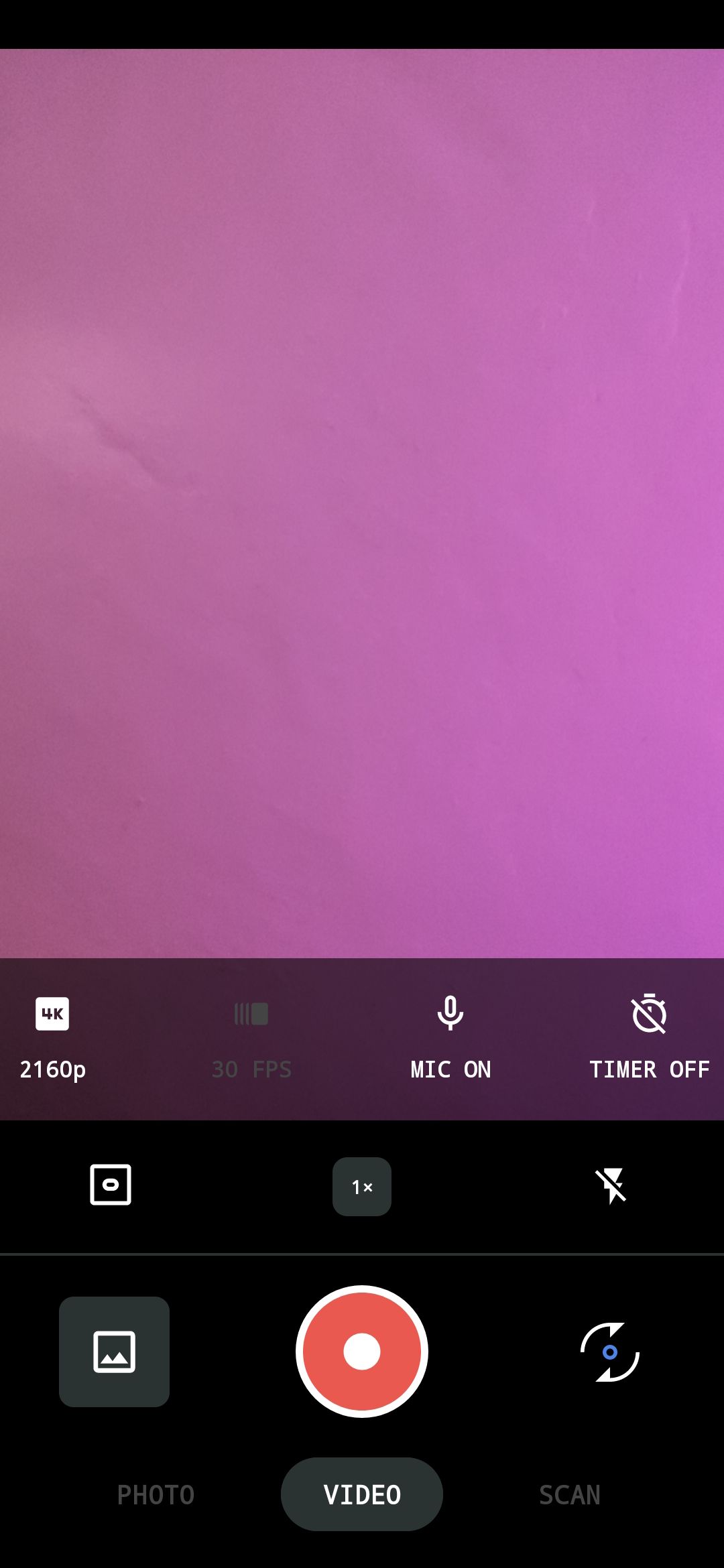This screenshot depicts a mobile device's video recording interface. The main screen is filled with a bright pink background, possibly indicating it is filming a pink piece of paper. The recording feature is active, as evidenced by the red record button. In a sub-menu, several settings are displayed: the video is being recorded in 4K resolution (2160p) at 30 frames per second, with the microphone turned on, indicated by the white 'Mic On' symbol. The timer function is disabled, denoted by the stopwatch icon with a slash. Below these, a small gray square marked with '1x' suggests the current zoom level. Additionally, the flash symbol crossed out with a diagonal line indicates the flash is off. At the bottom of the screen, there are three tabs labeled 'Photo,' 'Video,' and 'Scan.' The 'Video' tab is highlighted in light gray, signifying that the device is currently in video mode. The faint crease line visible in the pink background suggests that the subject being recorded could be a piece of pink paper with a fold.